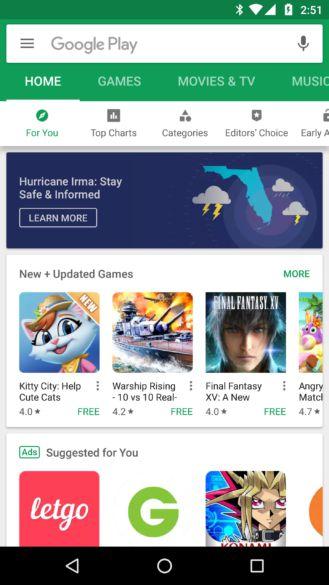A screenshot of the Google Play Store interface showcasing a white background with the main focus on the "Home" tab. At the top, a green header area features a search bar along with primary navigation tabs labeled "Home," "Games," "Movies and TV," and "Music." Within the "Home" section, the available options include "For You," "Top Charts," "Categories," "Editor's Choice," and "Early Access," with "For You" being the current active selection. 

Prominently displayed under "For You" is a banner with a notification message related to Hurricane Irma, advising users to "stay safe and informed" and offering a "Learn more" link, accompanied by an image of stormy clouds over Florida. Further down, the section highlights "New and Updated Games" such as "Kitty City," "Warship Rising," and "Final Fantasy XV," followed by a segment titled "Suggested for You" that includes the app "LetGo" among others, although the list is truncated in the image. The highlighted games vary in target audience, with some suitable for children and others appearing more appropriate for adults.